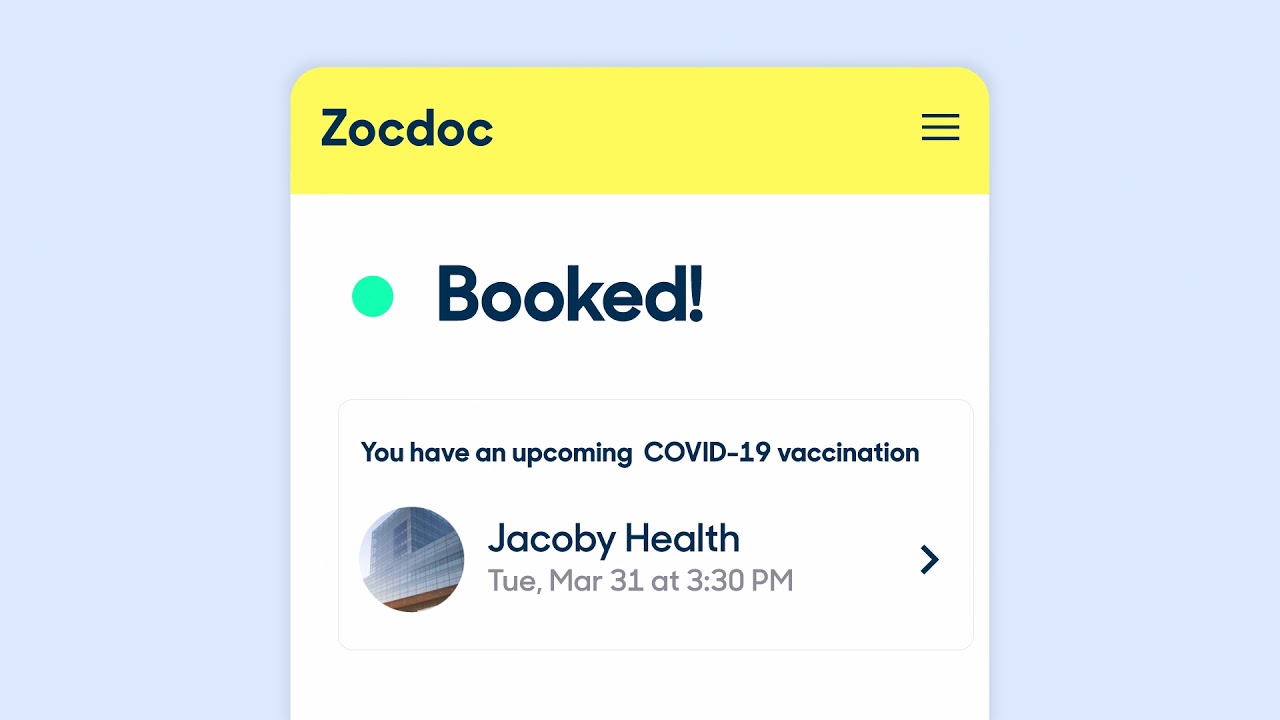Here's a detailed and cleaned-up caption for the image from the ZocDoc app:

The image depicts a ZocDoc app interface. The background features a horizontally situated blue rectangle. Within this rectangular space, a white box with a slight border of the blue background visible on the top is centrally positioned. This white box is topped by a yellow banner bearing the ZocDoc name "ZocDoc" in black font with a capital "Z" and the rest in lowercase. On the right side of this yellow banner are three small horizontal lines stacked vertically.

Below the yellow banner, there is a prominent white section. A green bullet point with the text "BOOKED!" in bold black letters is located here. Underneath this text is a thin gray line extending horizontally across the screen. Following this division, the text reads: "You have an upcoming COVID-19 vaccination."

Adjacent to this text is a circular image partially displaying blue and brown colors, likely depicting a building or an exterior structure. To the right of this circle, the text "JACOBY Health" is written in navy blue, followed by the details, "Tuesday, March 31st at 3:30 p.m." To the far right of this information, there is a right-facing navy blue arrow.

This detailed description provides a comprehensive visual of the ZocDoc app screen, emphasizing the important elements and layout for clarity.